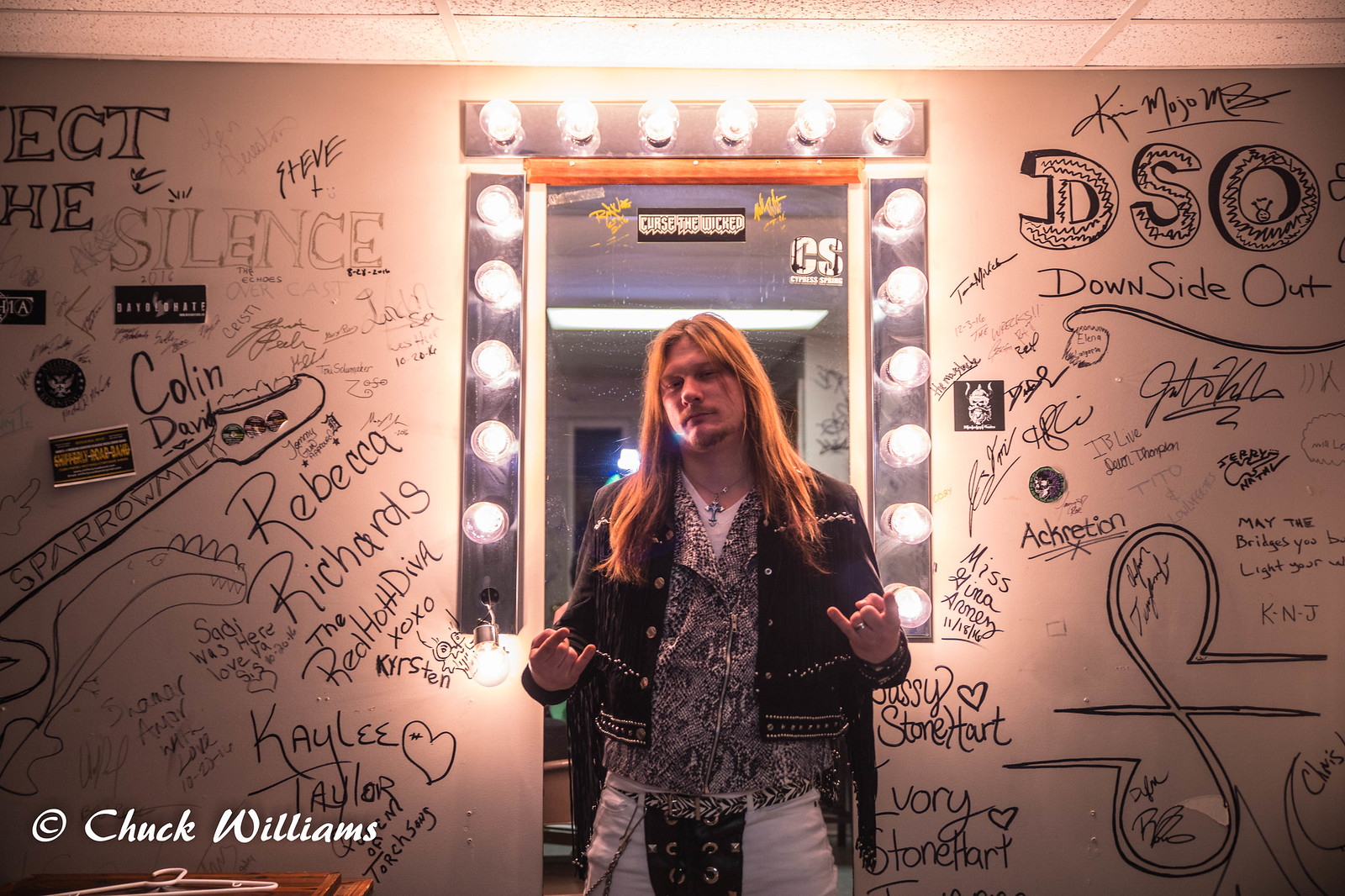This image captures a man who closely resembles Kid Rock, with long flowing blonde hair and a short goatee. He is dressed in a black jacket, possibly with an alligator pattern, layered over a white v-neck shirt and a gray vest, and is adorned with a blue cross necklace. The man, standing confidently with his hands raised in a rock and roll sign, is situated in what appears to be a dressing room. Behind him is a lit-up mirror with six white lights on the top and six on each side, though one light on the bottom left is hanging out of its socket. The surrounding walls and even the mirror itself are covered in a colorful array of graffiti and signatures, including names like Kaylee Taylor, Colin David, Sparrow Milk, Steve and the Silence, DSO, Downside Out, Accretion, and IB Live. A prominent copyright mark in the bottom left corner credits the photographer, Chuck Williams.